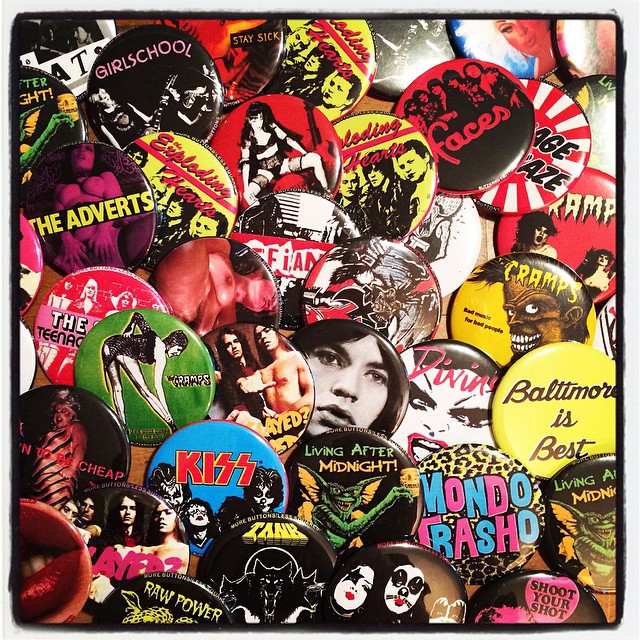This image features a close-up of a colorful collection of pin-back band buttons stacked on top of each other. These buttons, often seen adorning vests or backpacks, celebrate a medley of punk and metal bands. Among the vibrant assortment, prominent ones include multiple buttons for Kiss, showcasing the band members in their iconic makeup and logo, as well as several for The Cramps, featuring a skull-like character against a yellow backdrop. There are also buttons adorned with references to John Waters, such as one with a leopard print that says "Mondo Trasho," and another celebrating the drag actor Divine with the slogan "Baltimore's Best."

Mixed within this array are buttons for various other bands, including Tank, Slayer, Raw Power (Iggy Pop), The Adverts, and The Exploding Hearts. Some buttons also feature imagery from pop culture and horror films like Gremlins, while others bear more provocative images, such as nude women. Interspersed throughout are buttons with diverse color schemes — red, green, yellow — adding to the visual richness of the collection. The buttons are set against a background with a white, textured border that resembles a painted effect, which enhances their vintage appeal, suggesting that the collection is from the 1980s. The dense, overlapping layout of these buttons signifies a deep appreciation for the punk rock scene.